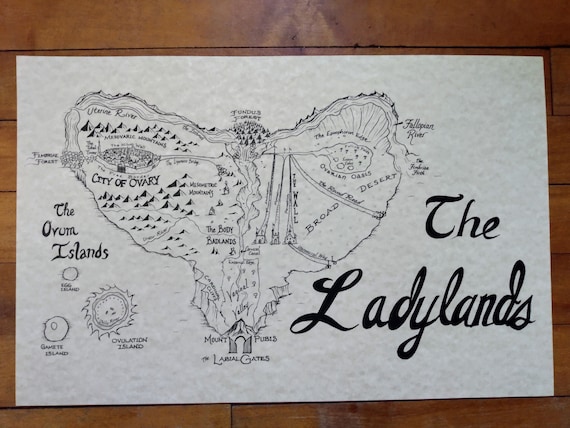A detailed map is depicted on a rectangular, slightly longer than tall, canvas set against a grayish-white background. The map, portraying the Ovum Islands, is placed upon what appears to be a wooden surface, potentially a floor or tabletop. The islands are drawn in a distinctive heart shape, with two lobes at the top tapering to a point at the bottom, reminiscent of the shape of female reproductive anatomy. 

Appropriately named "Ladylands," the map includes playful and suggestive labels like "Labinal Gates," "Mount Fumes," "Uterine River," and others, inferring a humorous, educational metaphor about female biology rather than an actual geographical location. The whimsical and slightly provocative nature of the names suggests the map serves as a teaching tool or a creative piece designed to evoke curiosity and perhaps a bit of amusement. The Ovum Islands are intricately detailed, making the map a curious blend of anatomical instruction and cartographic art.